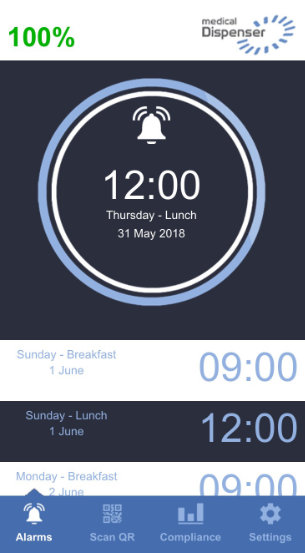The image features a medical dispenser reminder application. At the top right corner, the title "Medical Dispenser" is displayed in a smaller font above the word "Dispenser," which is larger, thicker, and in uppercase. The capital "D" in "Dispenser" incorporates a sideways circle at its end.

On the upper left side, a green font displays "100%". Below this, there's a dark blue rectangular box with a detailed light blue and white circular design. The design includes an inner light blue circle and a clock bell symbol at the center, which reads "12:00." Beneath this, the text "Thursday Lunch, 31 May 2018" is shown, indicating a specific scheduled reminder. Below this primary reminder, there are three additional alarm icons, suggesting multiple upcoming reminders.